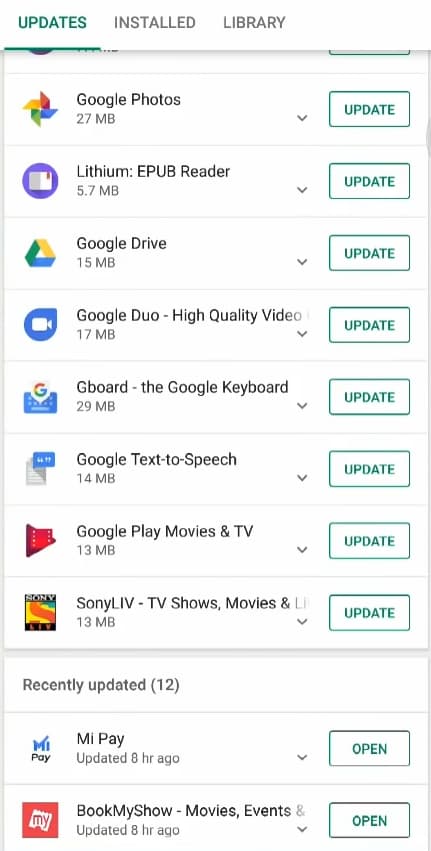The image displays a section titled "Updates" at the top, with three tabs underneath: "Updates" (highlighted in green with a green line beneath it), "Installed," and "Library" (both in gray). 

The list begins with "Google Photos," showing an update size of 27 megabytes. Adjacent to it is a dropdown menu, followed by a green-outlined button labeled "Update," consistent throughout for all listed apps. 

Next is "Lithium: EPUB Reader" with an update size of 5.7 megabytes, accompanied by the same dropdown menu and "Update" button. 

Following this, the list includes:
- "Google Drive" (15 megabytes), "Update" button 
- "Google Duo: high-quality videos" (17 megabytes), "Update" button 
- "Gboard: the Google keyboard" (29 megabytes), "Update" button 
- "Google Text-to-Speech" (14 megabytes), "Update" button 
- "Google Play Movies & TV" (13 megabytes), "Update" button
- "Sony LIV-TV, Shows and Movies" (13 megabytes), "Update" button

At the bottom, a section labeled "Recently Updated (12)" is visible, showing "My Play" as updated eight hours ago with an "Open" button next to it.